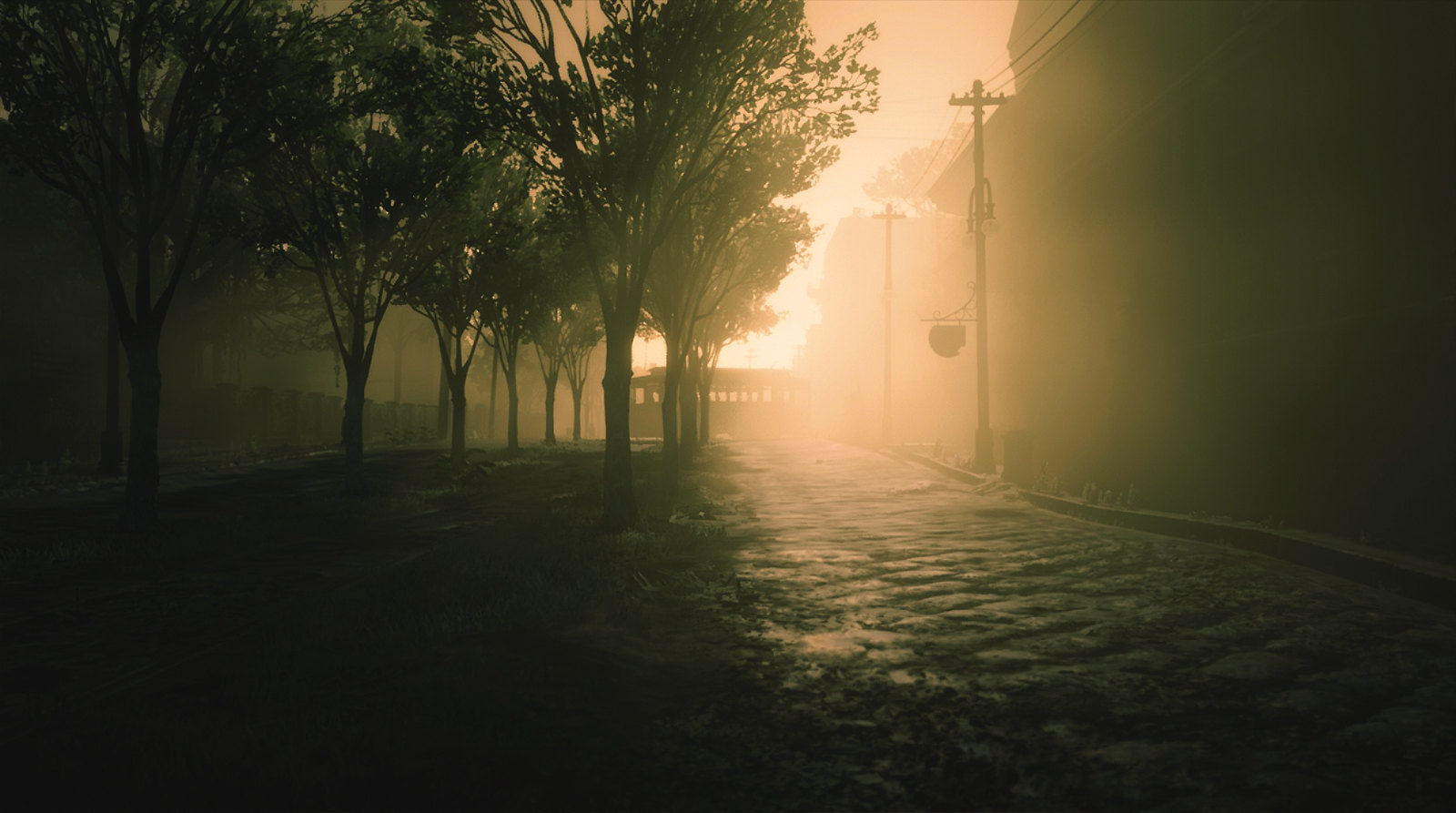This photograph captures a tranquil and mysterious scene, set in what appears to be an alleyway or walkway paved with stone. Small, decorative trees line the left side of the path, adding a gentle touch of nature to the otherwise urban setting. The stone walkway itself appears rippled, possibly covered in a thin layer of water that reflects the ambient light. On the right side in the background, a row of power poles stand tall against a smoky haze that envelops the entire scene, giving it an ethereal and surreal quality. A bright pink light glows intensely in the background, casting a radiant beam down the walkway and contributing to the otherworldly atmosphere. On the right, a fence runs parallel to the path, leading the eye toward the silhouetted forms in the distance. In the center of the composition, far in the background, a structure with numerous windows looms, its details obscured by the haze but still adding a hint of urban sprawl to the scene.